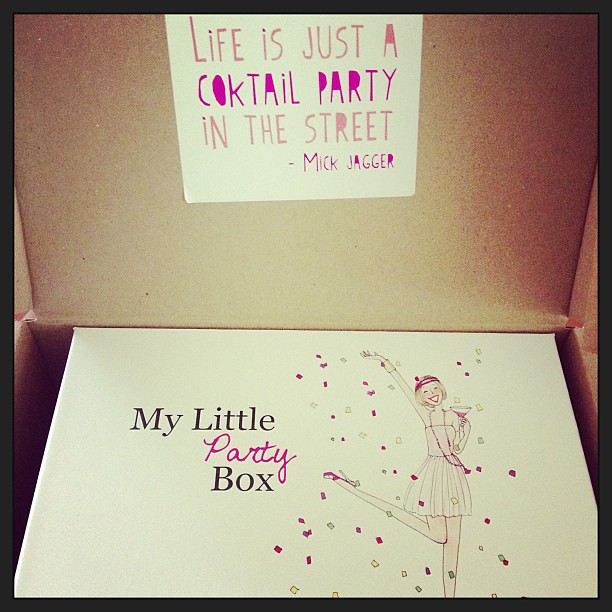This colored photograph showcases a festive scene centered around a pair of nested boxes. The outer container is a brown cardboard box, its lid adorned with a handwritten quote in pink ink that reads, "Life is just a cocktail party in the street" — attributed to Mick Jagger. Upon opening this outer layer, one finds a smaller, white party box inside. This white box features a lively illustration of a young woman dressed in a pink dress and high heels, wearing a beret, and holding a glass of champagne. Her jubilant pose, with one leg kicked up, captures the essence of celebration, as multicolored confetti in shades of yellow, red, purple, and green surrounds her. In bold font, the words "My Little Party Box" are prominently displayed, with 'party' highlighted in pink and capitalized. The image conjures a sense of joy and festivity, with the vibrant scene encapsulated within the nested boxes.